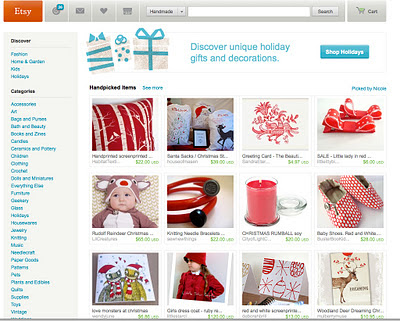The image depicts the homepage of the Etsy website. In the top left corner, the site's name "Etsy" is prominently displayed in white text against an orange background. Centered at the top, there is a search bar for users to explore various listings. On the top right, an icon shaped like a shopping cart signifies the user's cart.

The main section of the page features an advertisement banner promoting holiday shopping. The banner's text, "Discover unique holiday gifts and decorations," is presented in blue, placed next to images of gift bags in shades of gray and blue on the left. To the right of this message, a blue button reads "Shop Holiday."

Below the banner, a section labeled "Hand-picked items" showcases a diverse array of products. Though the product names are blurred and unreadable, a variety of items are depicted, including pillows, shoes, candles, cables, toddler clothes, and paintings. The dominant colors of the products are red, white, and pink.

On the left side of the webpage, a vertical menu lists various categories for browsing. These include "Discover," "Fashion," "Home and Living," "Holidays," as well as other categories like "Accessories," "Art," "Bags and Purses," and "Bath and Beauty." Some of the category names are partially visible due to the limited clarity of the image.